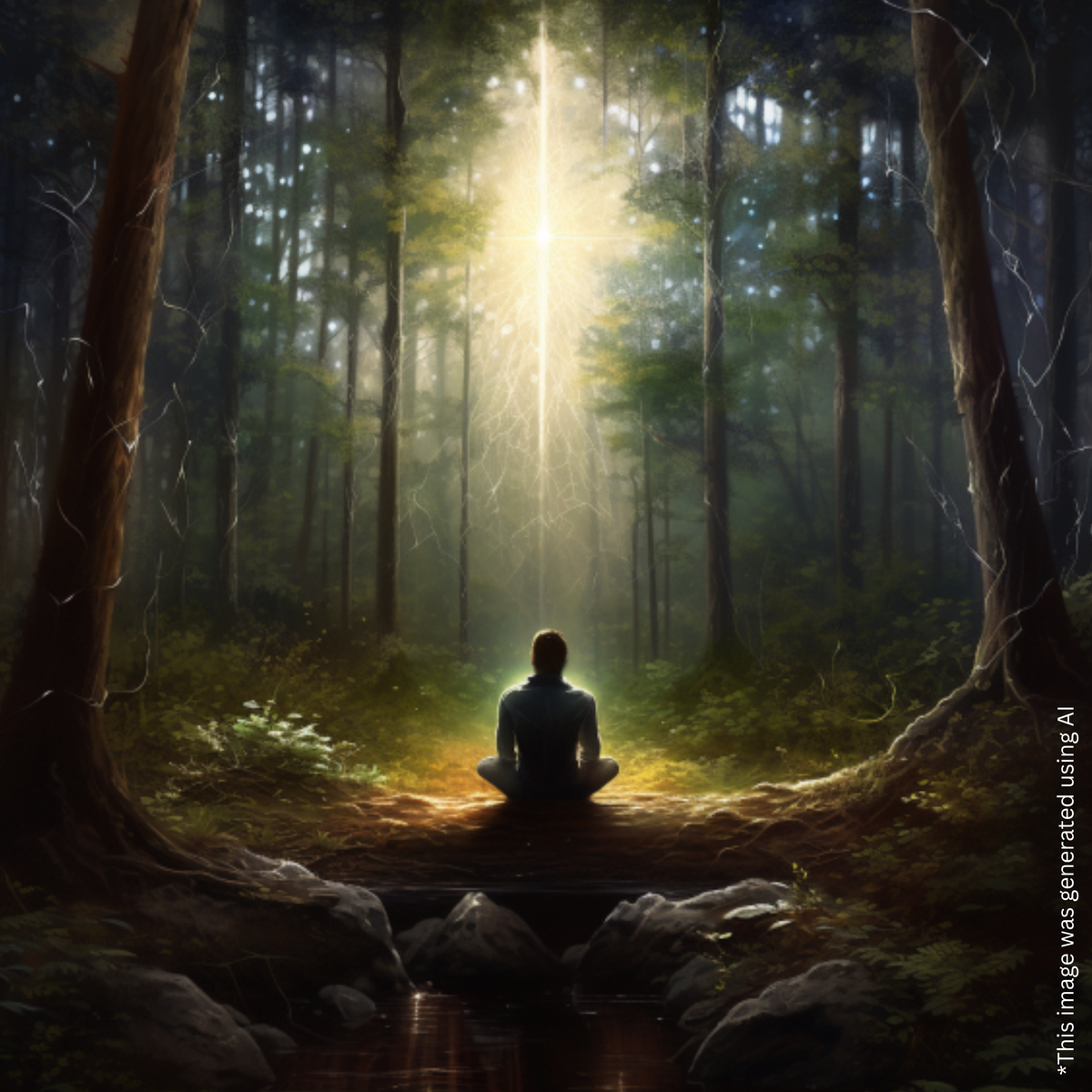This AI-generated image, as noted by the vertical white text on the bottom right, depicts a human figure sitting cross-legged on a fallen log in a lush, evergreen forest. The figure, whose back faces the camera rendering them androgynous with wide shoulders and short hair, is silhouetted against a striking beam of white light. This powerful beam, originating from a point obscured by the treetops, extends vertically to illuminate the shoulders of the figure and the surrounding forest. The scene is dominated by greenery with tall pine trees and dense ground cover, while rocks and a stream are visible behind the log. The ethereal light creates an almost heavenly glow, contrasting starkly with the darkened foreground, casting an awe-inspiring atmosphere.